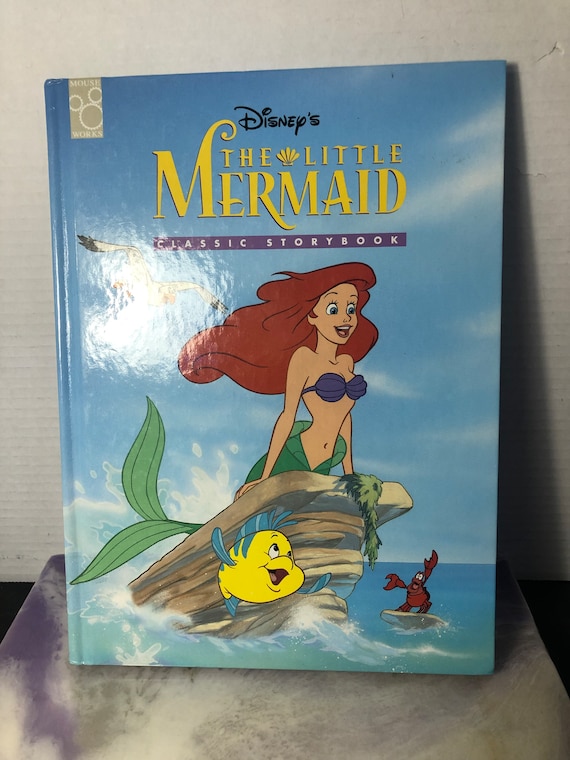In this indoor photograph, a large, hardcover edition of Disney's "The Little Mermaid: Classic Storybook" is prominently displayed, leaning against a white wall on a table. The book's predominantly blue cover features a picturesque scene where a red-haired Ariel, adorned with purple shell bra, perches on some rocks with her green fins elegantly draped. The background portrays a gradient blue sky blending into a darker blue ocean, with wispy clouds and a seagull soaring above, adding to the whimsical feel. Nearby, a cheerful yellow fish leaps out of the lighter blue waters while Sebastian the lobster, often mistaken for a crab, appears jovially positioned in the water below Ariel. The scene, filled with joyful expressions and vibrant colors like yellow, red, teal, and dark blue, radiates a sense of happiness and rejoicing among the characters. Additionally, a purple rectangle beneath the title clearly labels it as a "classic storybook," emphasizing its timeless charm.